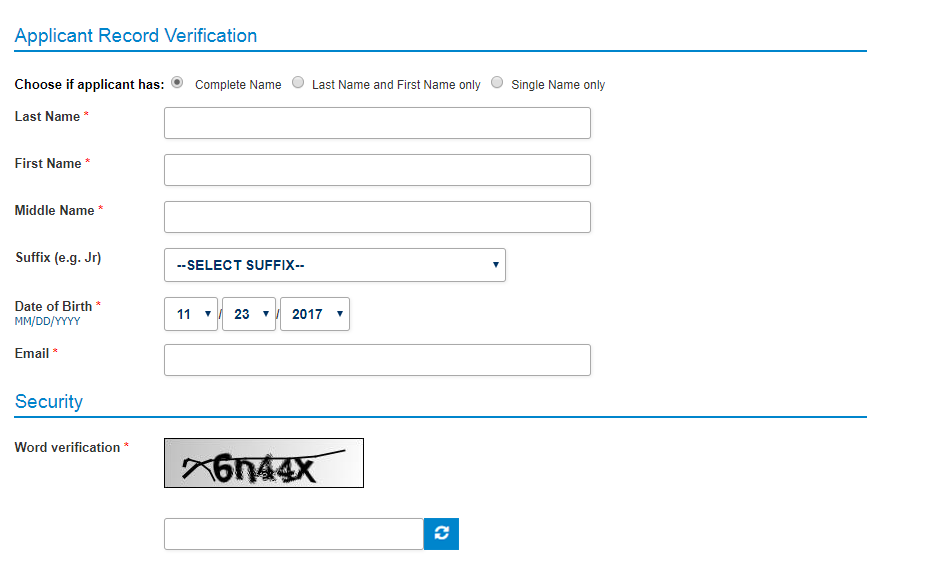The image captures a web page designed for applicant record verification. At the top left corner, the page is titled "Applicant Record Verification" in blue text, with a blue horizontal line running directly beneath it. The main body of the page is set against a white background. 

At the top of the body section, there are multiple options for selecting the applicant name information. The options are radio buttons labeled: "Complete Name," "Last Name and First Name Only," and "Single Name Only," with "Complete Name" already selected. 

The subsequent part of the page contains detailed input fields necessary for the verification process. Each of these fields includes a red asterisk, signifying that they are mandatory. The text boxes for "Last Name," "First Name," and "Middle Name" appear first, followed by a dropdown box for selecting a suffix to the name. Below these fields, there is a date of birth entry, which is currently filled out with the date "11-23-2017." 

Additional mandatory fields include a text box for "Email" and a security field for verification, labeled "Captcha." The page concludes with a prominent blue button for submitting all the entered information once the captcha is correctly filled in.